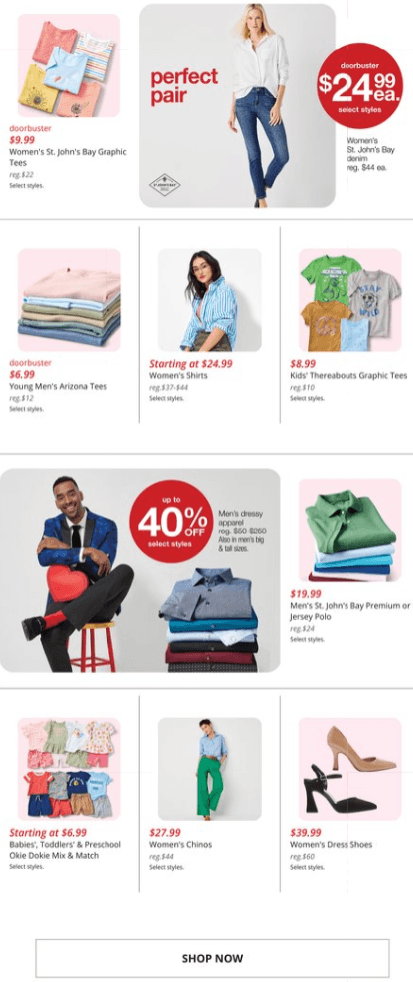A screenshot from a mobile device captures a shopping webpage displaying various items for sale, arranged in four distinct rows. The first row features an image of a woman wearing a white shirt and denim pants, with the text "Perfect Hair" written in red to her left. To her right, a red circle displays the price, "$24.99 each," in white text. The second row showcases a mix of clothing items: the first image features folded t-shirts, the second image shows a woman in a blue shirt, and the third image displays four t-shirts in green, gray, brown, and blue. The third row presents a man seated, dressed in a blue jacket, white shirt, black pants, and red socks.